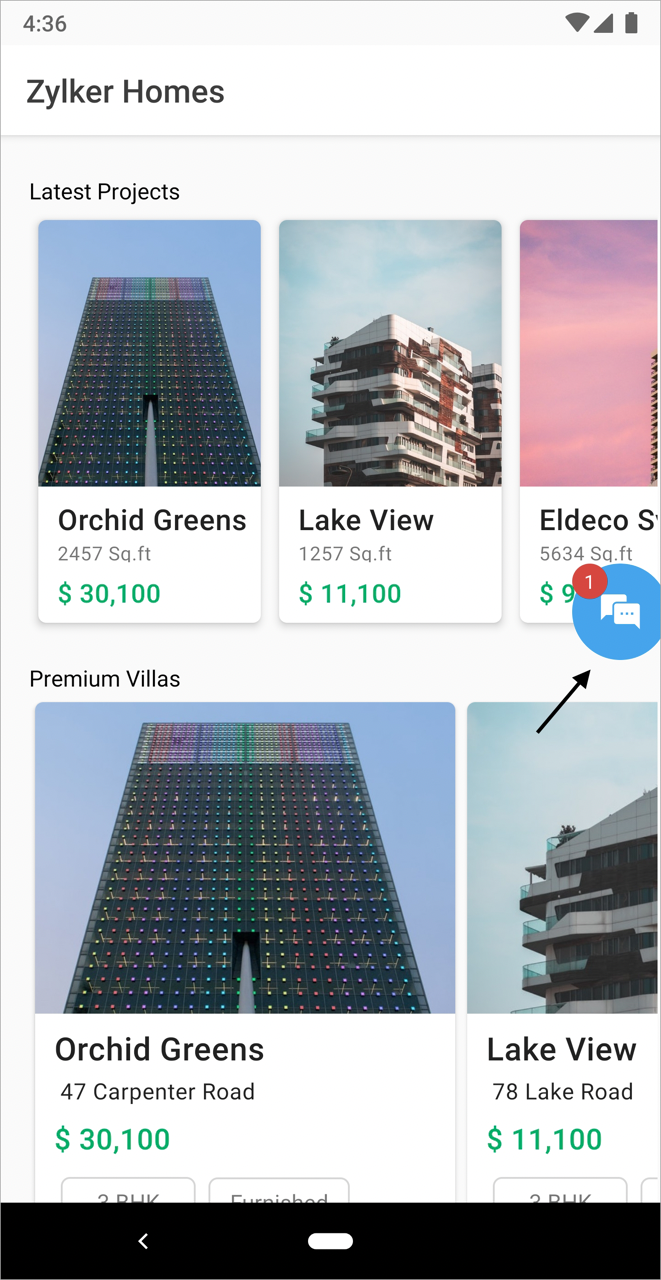The image features a detailed interface of a real estate listing platform, showcasing properties by "Zilker Homes" (styled as "Zylker Homes").

1. **Timestamp**: Located at the top left corner, "4:36" is printed in dark gray on a light gray background.
2. **Banner**: Beneath the timestamp, a white banner displays "Zilker Homes" in bold black letters.
3. **Background and Icons**: Following the banner, the background transitions to light gray, populated with various icons representing different properties.

### Property Listings:
- **Property 1: Orchid Greens**
  - **Icon**: Features a large building with a rainbow tint.
  - **Title**: "Orchid Greens" in bold black lettering.
  - **Details**: 
    - Size: "2,457 sq. ft." in light gray lettering.
    - Price: A green bold dollar sign followed by "30,100" (formatted as "$30,100").

- **Property 2: Lake View**
  - **Icon**: Shows another building.
  - **Title**: "Lake View" in bold black lettering.
  - **Details**: 
    - Size: "1,257 sq. ft." in light gray lettering.
    - Price: "$11,100" in bold.

- **Property 3: El Deco**
  - **Title**: Partially visible, labeled "El Deco" (title cut off).
  - **Details**: 
    - Size: "5,634 sq. ft." in light gray lettering.  

### Additional Elements:
- **Messaging Notification Icon**: Overlayed toward the right side of the El Deco property listing. It's a circular blue icon with two messaging symbols and a red notification badge with a white "1" at the top left, indicating a new message.

### Enhanced Visuals:
- **Larger View of Orchid Greens**:
  - Positioned at the bottom, providing a more detailed view of the property.
  - Overlaid with the text "Premium Villas" at the top.

- **Larger View of Lake View**:
  - Situated to the right of the Orchid Greens larger view, signaling a transition into the Lake View property details.

This comprehensive interface connects potential buyers with detailed real estate options, blending visuals with essential property information.